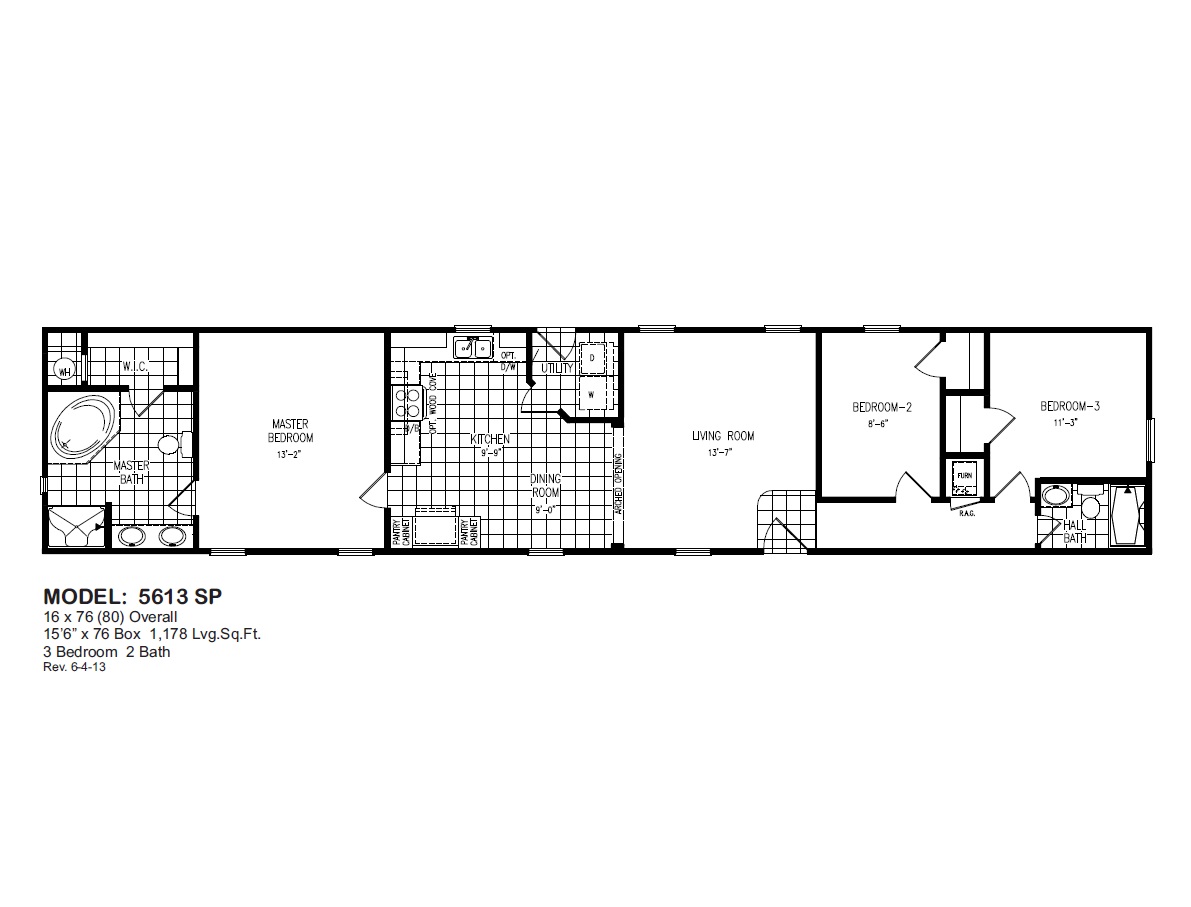This detailed architectural floor plan illustrates the layout of Model 5613SP, a home measuring 16 feet by 76 feet overall. Located at the bottom left of the plan is a label containing essential details: Model 5613SP, dimensions of 16 by 76 feet, a configuration of three bedrooms and two bathrooms, and a revision date of June 4, 2013. The plan is presented as a long horizontal rendering in black and white with black text on a white background.

The layout from left to right begins with the master bath, which is connected to the master bedroom. Adjacent to the master bedroom is the kitchen, followed by the dining room. Continuing to the right, the plan features a spacious living room. Further to the right, you find bedroom two, and finally, bedroom three at the farthest right end of the layout. Each room is arranged in a straight line, providing a clear and efficient flow through the house.